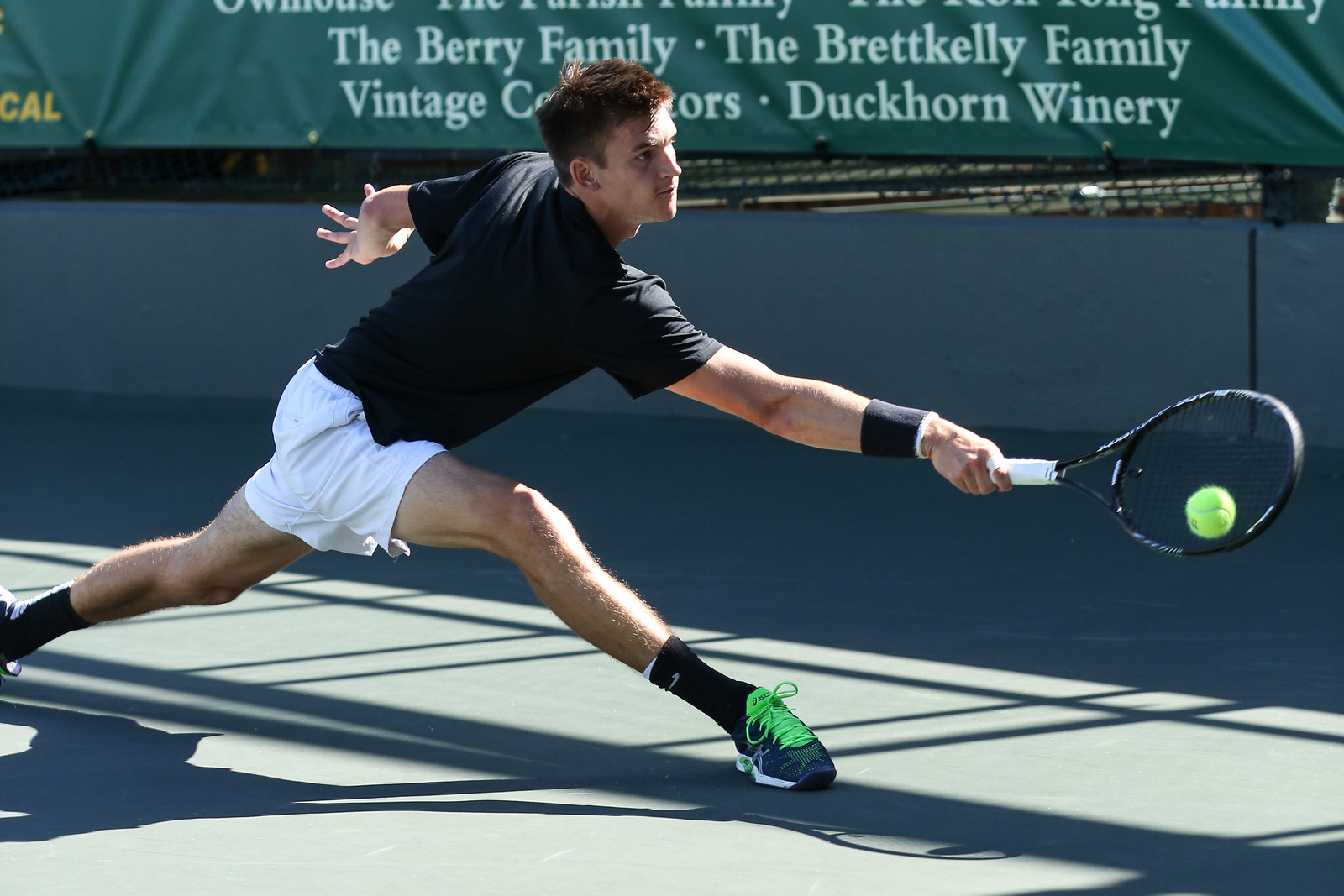In this photograph, a tennis player is captured in mid-action on a tennis court, frozen in a dramatic stretch with both arms fully extended as he reaches to hit a tennis ball with his racket. His right arm wields a racket with a black frame and a white handle, while his eyes intensely focus on the imminent contact with the green ball. His left hand mirrors his right, stretching out to maintain balance. He wears a black t-shirt, white shorts, and green-laced shoes. His stance is extraordinary, with legs splayed in a near-split position, indicating the extreme effort to reach the ball. The court itself has a distinct green hue, matching the player's shoelaces. Behind him, a concrete wall is adorned with a green banner featuring advertisements from sponsors such as the Barry Family, Bretko Lee Family, Vintage (partially cut off), and Duckhorn Winery. This rich, detailed image captures the athleticism and intensity of a tennis match.